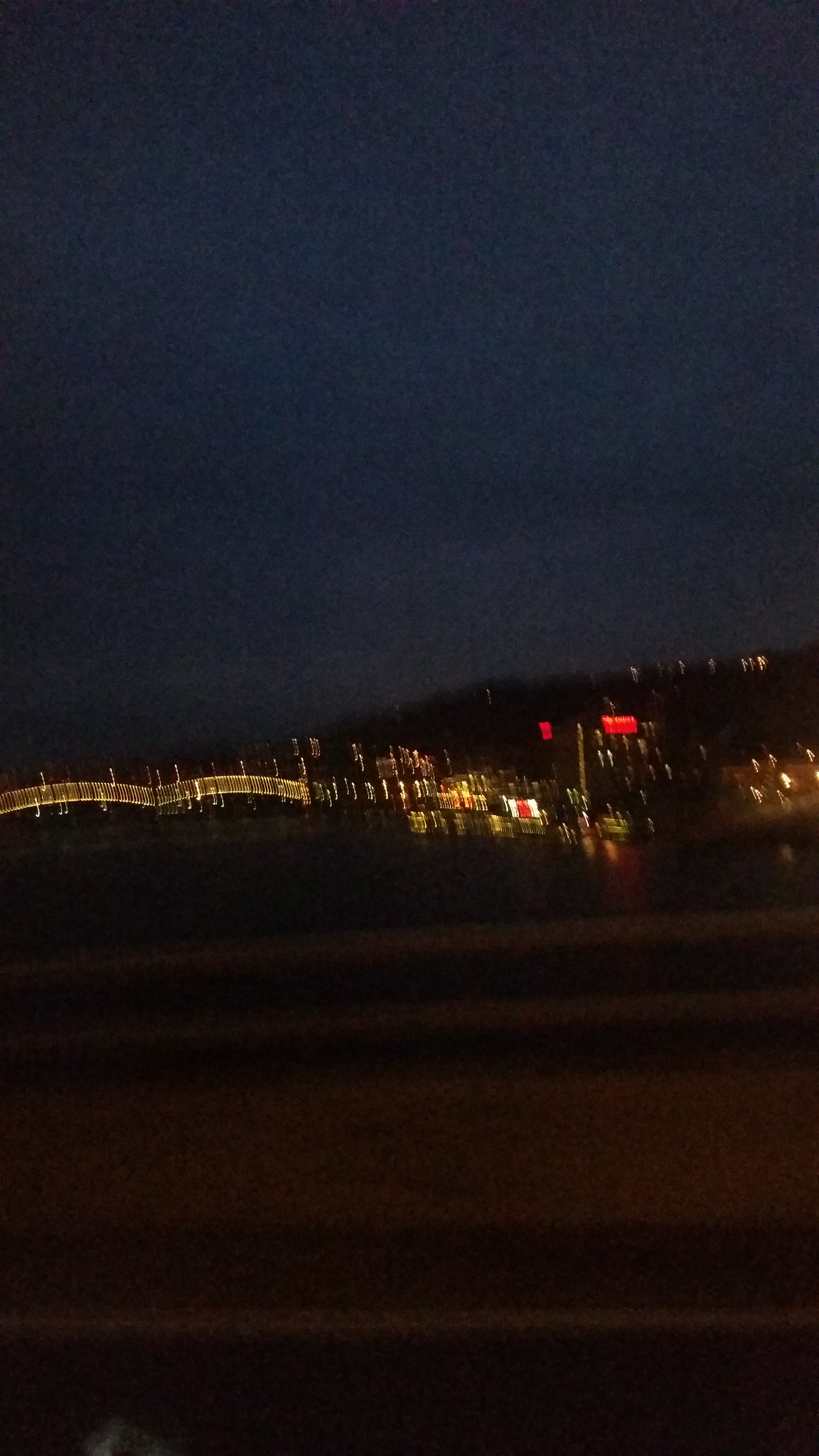The photograph, taken from an elevated vantage point such as a hillside or mountain, captures a distant city at night. The city’s twinkling lights, a mixture of neon and white, stretch across the center of the image, reflecting faintly on what appears to be water in the foreground, suggesting a harbor or pier. The dark, bluish sky frames the backdrop, adding to the nocturnal ambiance. The lower section of the image is mostly black, likely due to shadows from the hillside or the car in which the photographer was traveling, as suggested by the presence of a guardrail, road markings, and a possible wing mirror. Despite the slight motion blur and overall darkness, the glowing hillside city and hints of infrastructure like a bridge are clearly discernible, providing a captivating contrast against the serene, dark expanse.